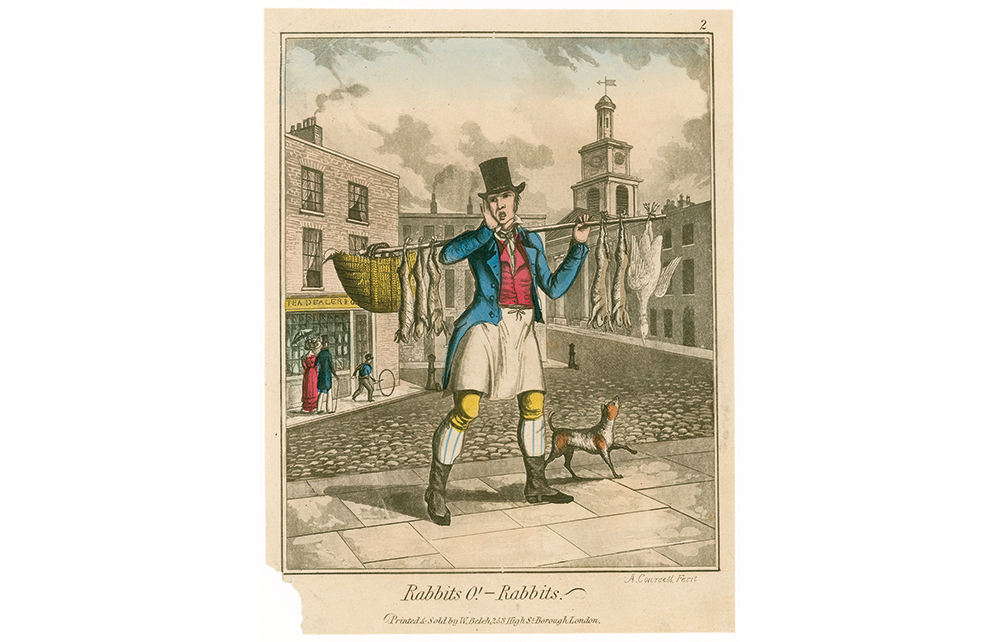In this old, light brown-tinted drawing, possibly a page from a Victorian-era book or magazine (noted by the number "2" in the top right corner), we see a merchant from the late 1800s or early 1900s standing on a cobblestone street in London. Dressed in short white pants, yellow trousers, tall striped socks, a white apron or skirt, a blue coat with tails, a red vest, and a black top hat, the man is holding a long stick across his shoulders. Hanging from the stick are several dead rabbits—three on one side and two with a goose on the other—indicating he is likely selling rabbit skins or meat. He also carries a basket, and there's a dog walking near him, possibly his companion. The image captures a bustling city scene with people moving along the sidewalks in front of stone buildings, where only the people's colorful clothing stands out against the otherwise colorless background. A yellow sign is visible in the distance, and the bottom of the image reads, "Rabbits O' Rabbits," suggesting the man's trade.